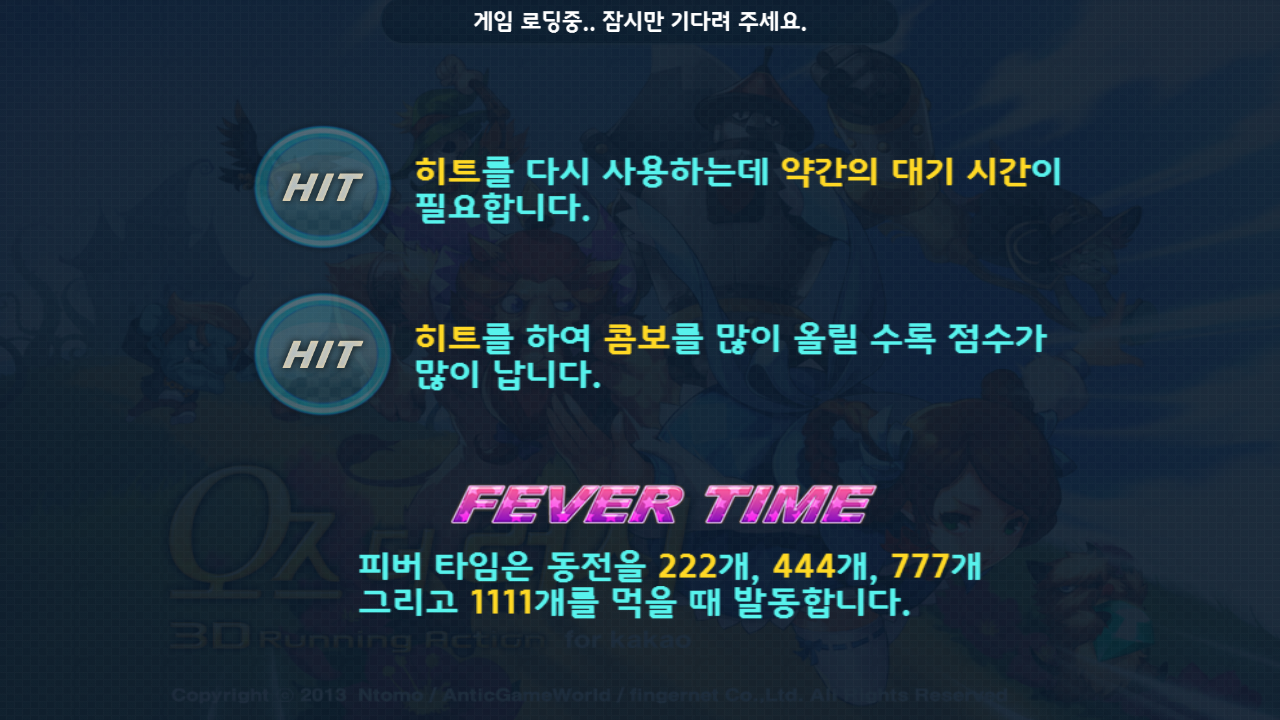The image depicts a visually captivating scene reminiscent of a video game interface, featuring a blend of vibrant text and dynamic anime-style graphics. In the background, there is a blurred cartoonish setting with various 3D characters, including a woman, a lion, and a robot, engaging in running action within a sky backdrop. This backdrop is labeled with text such as "3D running action for Kakao," "Copyright 2013 Natomo, Antic Game World," and additional blurred content that hints at a dynamic, playful graphic design.

At the forefront, the most eye-catching elements are two round blue circles on the left side, each prominently displaying the word "HIT" in white. Above and below these circles, there's Asian writing, which might be in Mandarin, Korean, or another Asian language. Centered below the "HIT" circles, the phrase "Fever Time" appears in bright pink, flashy neon-style letters, further contributing to the energetic and engaging visual. Below "Fever Time," there is another sentence in the same Asian language, adding to the layered complexity of the image. The overall color scheme of the image is predominantly navy blue, which frames the vivid text and characters, making them stand out even more effectively.